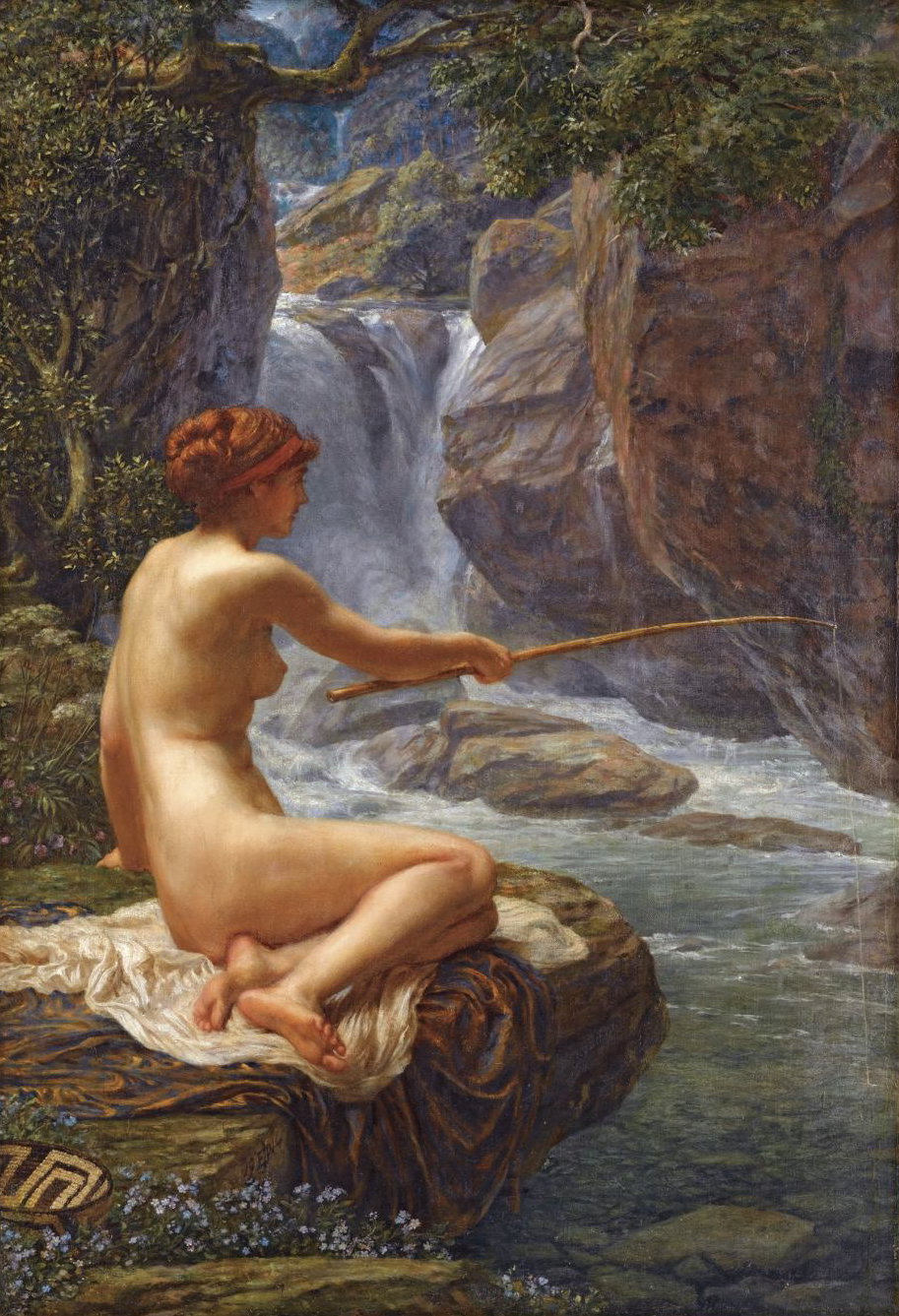This painting, evocative of the early 1800s, portrays a serene yet striking scene of a naked woman fishing near a waterfall. Bathed in natural light, she is positioned on the edge of a cliff, seated on a white satin sheet that overlays a brown blanket. The woman's red hair is intricately pinned up, adorned with a red headband, emphasizing her fair skin. She faces slightly backward, allowing a view of her stomach and right breast, while her knees are bent and tucked to her right. In her right hand, she holds out a rudimentary fishing rod, a simple stick with a line dipping into the clear, shallow water beneath her, which deepens as it flows away.

Her surroundings contribute to the romantic atmosphere: the vigorous waterfall cascades in the background, framed by rocky cliffs on either side. A tree with a brown trunk and small green leaves extends over the entire top part of the painting, enhancing the lush natural setting. Nearer to the woman, purple flowers grow, adding splashes of color, and at the bottom left, there is a basket with an elaborate black and white woven pattern. The area is dotted with small blue flowers, completing this tranquil and picturesque tableau.